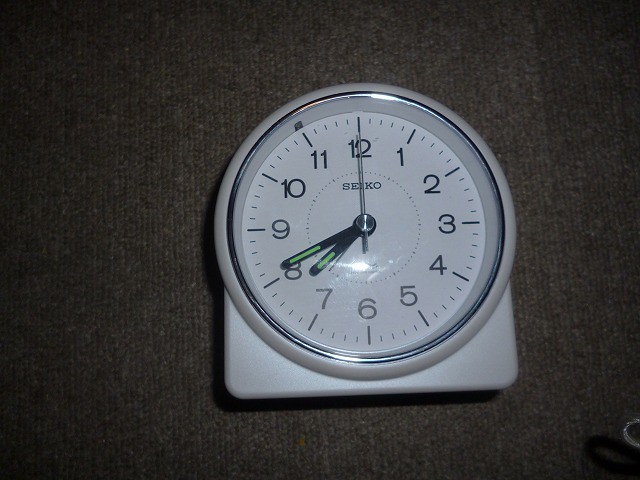The image captures a small white clock placed on a typical beige carpeted floor commonly found in office settings. The clock features traditional black hands with distinctive green lines running through them. Both clock hands are pointing to the eight. In the bottom right corner of the image, there is a partially visible object, possibly a chair leg or a purse loop, casting a shadow. The scene suggests an everyday office environment accentuated by the presence of the clock lying on the carpet.